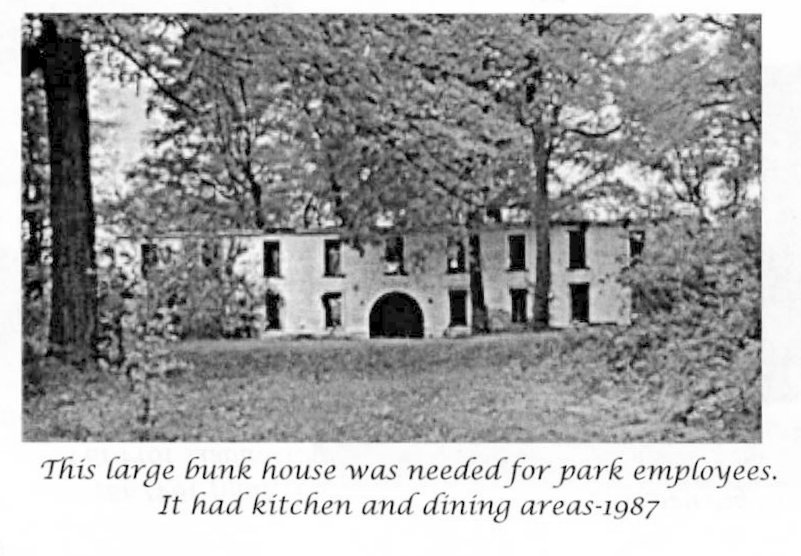This black-and-white photograph depicts a sprawling, two-story bunkhouse surrounded by dense foliage. The prominent structure features numerous windows on both levels and a distinct arched entrance on the ground floor. The ground before the building is covered in grass, while trees frame the house on all sides, with their leaves partially obscuring the second-story windows. A particularly prominent tree trunk dominates the left-hand side of the image. Below the photo, a caption in cursive reads: "This large bunkhouse was needed for park employees. It had kitchen and dining areas - 1987." The photo’s composition emphasizes the overgrown, natural setting of the building, highlighting its historical context and function in a park environment.